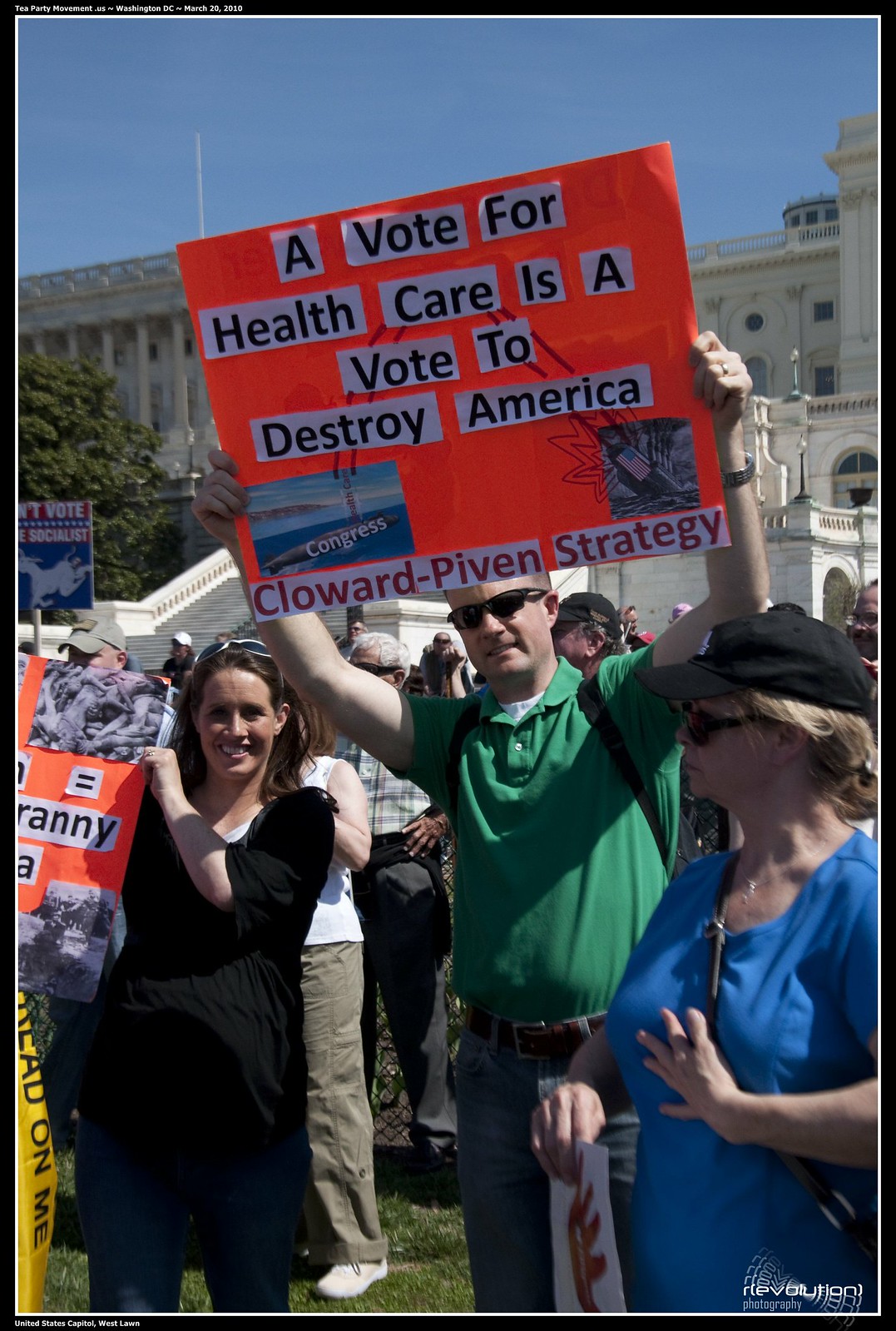The image captures a protest seemingly directed against Obamacare or socialized healthcare, prominently featuring three individuals in front of what appears to be a courthouse with tall, white columns and visible steps on the left-hand side. Central to the image is a man in a green shirt, dark sunglasses, and dark pants, holding an orange poster with black lettering that reads, "A vote for healthcare is a vote to destroy America," followed by "Cloward-Piven strategy" in red below. To his left stands a woman in her late twenties, smiling, holding another orange poster partially obscured by the frame, but the visible text reads "tyranny." She wears a black shirt. On his right, a woman in profile, wearing a blue dress, a black baseball cap, and sunglasses, is holding an unreadable sign. Behind this trio, other protesters are milling around and engaging in conversation, adding to the bustling atmosphere of the protest.